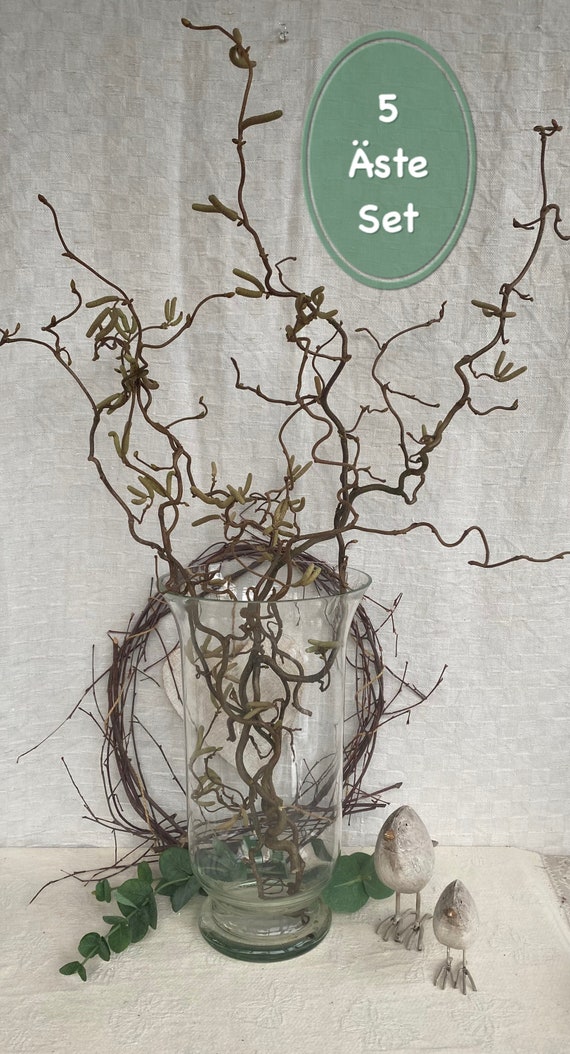The image features a detailed arrangement set against a backdrop of white linen sheets, with a woven blanket covering the surface. At the center, there is a tall, clear glass vase with a bell-shaped opening that fans out at the top. Inside the vase, there are several thin, gnarled branches that extend upward, noticeably devoid of leaves but dotted with cylindrical growths that could be seed pods. The plant inside the vase appears dry and lifeless. Beside the vase, there is a small green branch with fresh leaves, not connected to the plant inside. To the right of the vase, there are two handcrafted stone birds, each styled to resemble small eggs with legs and drawn-on faces. The entire arrangement is placed carefully, giving a delicate yet artistic impression.